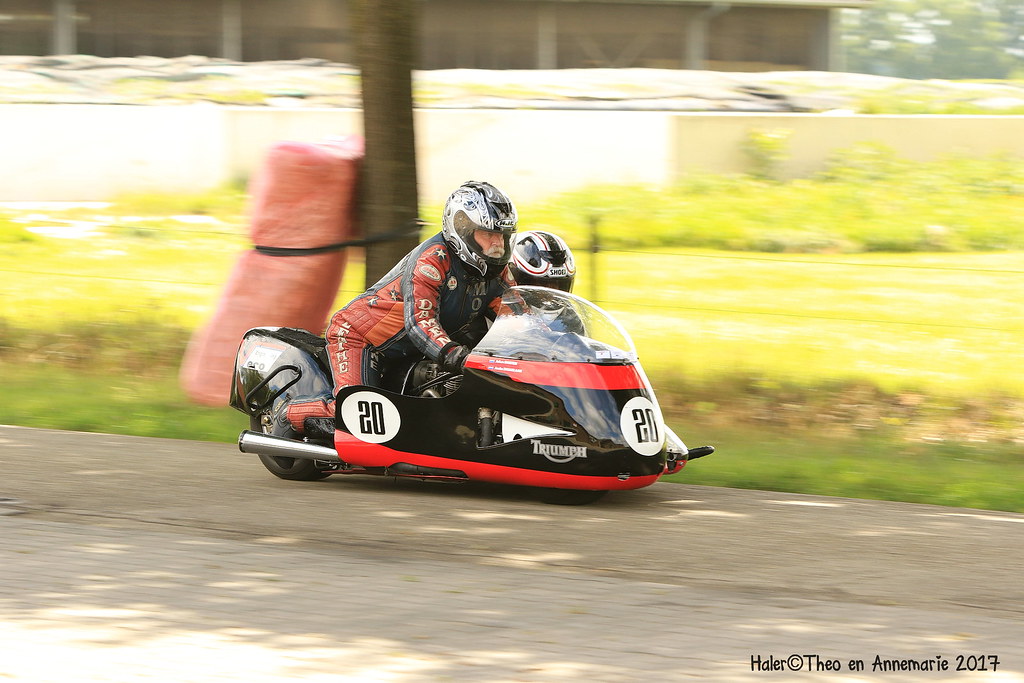In this image, a very small, black motorcycle, which closely resembles a go-kart due to its low profile and compact size, is seen speeding along a blurred background of green brush, grass, and a tree adorned with something red tied around it. The motorcycle, marked with the number 20 on both the front and side, prominently displays the Triumph logo, reinforcing its identity as a Triumph bike. It features a silver exhaust with a distinctive red line circling it and a clear windscreen at the front. The scene captures two individuals; the driver, a man sporting a mustache and beard discernible through his helmet's visor, is clad in a red jumpsuit with text along the side. Both riders wear helmets, with the second passenger's only visible feature being their helmet. The image is slightly blurry, conveying the sense of speed and motion. At the bottom right corner of the photograph, the text "Hailer, copyright, Theo, Anne-Marie, 2017" is inscribed, further authenticating the image. The driver appears taller, emphasizing the dynamic and thrilling nature of the ride.